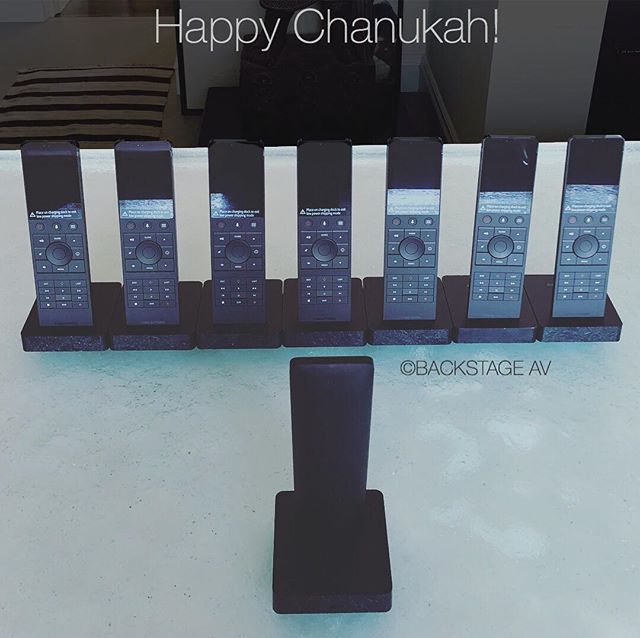This image presents a promotional display with a festive theme, featuring a neat row of seven remote controls, each positioned vertically on black, stone-like bases. The remotes are lined up against a backdrop of an office space, evident by hints of furniture like what seems to be a metal file cabinet. Above the display, the phrase "Happy Chanukah" stands out in celebratory white text. One unique remote control faces this array, standing alone on a similar black base, creating a focal point within the setup. The entire arrangement rests on a grey and white table, possibly resembling a concrete surface. Below the devices, the text “Copyright Backstage AV” acknowledges the display’s origin, printed in black on the base, contributing to the professional aesthetic of the advertisement.